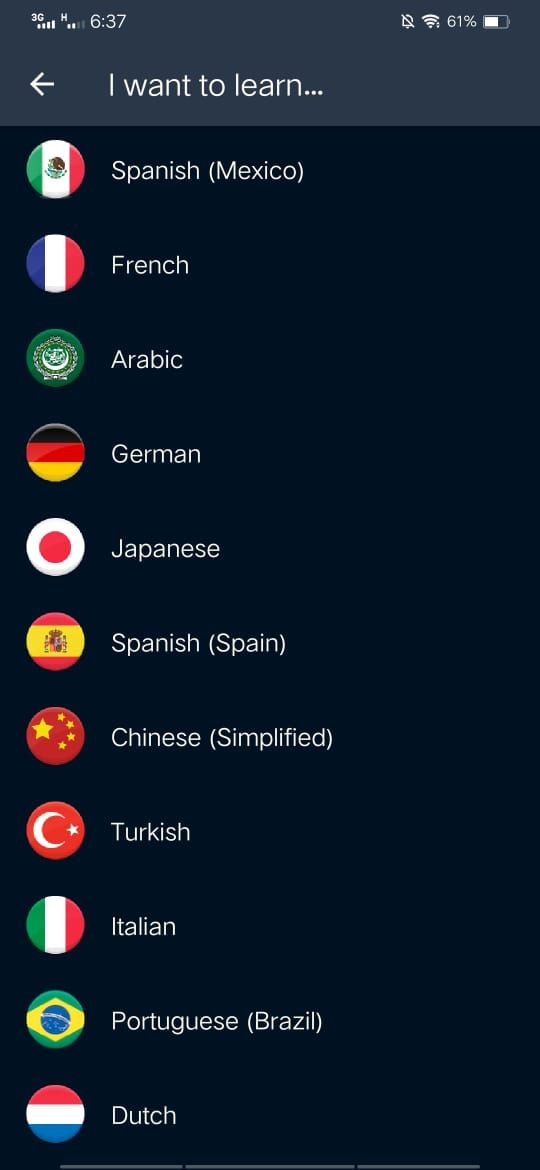The image is a detailed screenshot of a mobile application or website interface captured on an Android device, recognizable by its distinctive UX/UI design. The top status bar on the screen displays various indicators including the time at 6:37, mobile data connectivity (potentially 5G or 3G), a Wi-Fi connection, and a battery level at 61%, alongside several notification icons.

Beneath the status bar, the header of the page prominently features the text "I want to learn," accompanied by a back arrow for navigation purposes. Below this header, the main body of the screen showcases an array of language options, each represented with their respective national flags. The languages and their respective countries/flags displayed include:

- Spanish (Mexico) with the Mexican flag
- French with the French flag
- Arabic with the flag from an Arabic-speaking nation
- German with the German flag (black, red, and yellow horizontal stripes)
- Japanese with the Japanese flag (a red circle on a white background)
- Spanish (Spain) with the Spanish flag
- Chinese (Simplified) with the Chinese flag
- Turkish with the Turkish flag
- Italian with the Italian flag
- Portuguese (Brazil) with the Brazilian flag
- Dutch with the Dutch flag

Each language option is visually distinguished by its corresponding country’s flag, making it easy for users to identify and select their desired language preferences.